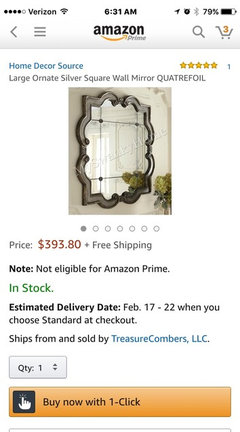A screenshot from a cell phone displaying an Amazon.com page. The top section features a black status bar against a white background, indicating a Verizon network with four out of five bars, full Wi-Fi signal, the current time of 6:31 AM in the center, and an active GPS icon on the right. Bluetooth is turned off, and the battery is at 79%.

Below the status bar, the interface shifts to a gray background with a back arrow on the left and several icons. The Amazon Prime logo is centered, flanked by a magnifying glass search icon and a shopping cart containing the number three in green.

The product shown is described as "Home Decor Source," and it has received five yellow stars based on one review. The item listed is a large, ornate silver square mounting mirror from a portfolio. The image displays a fancy-looking dark wood mirror mounted on a white wall. 

The price is listed in gray text with a red price tag of $393.80, plus free shipping. The product is not eligible for Amazon Prime. Availability is marked in green as "In Stock," with an estimated delivery date of February 17th through 22nd for standard shipping. The item is shipped and sold by Treasure Combers, LLC.

The section ends with a quantity selection set to one and a prominent orange "Buy Now with 1-Click" button.